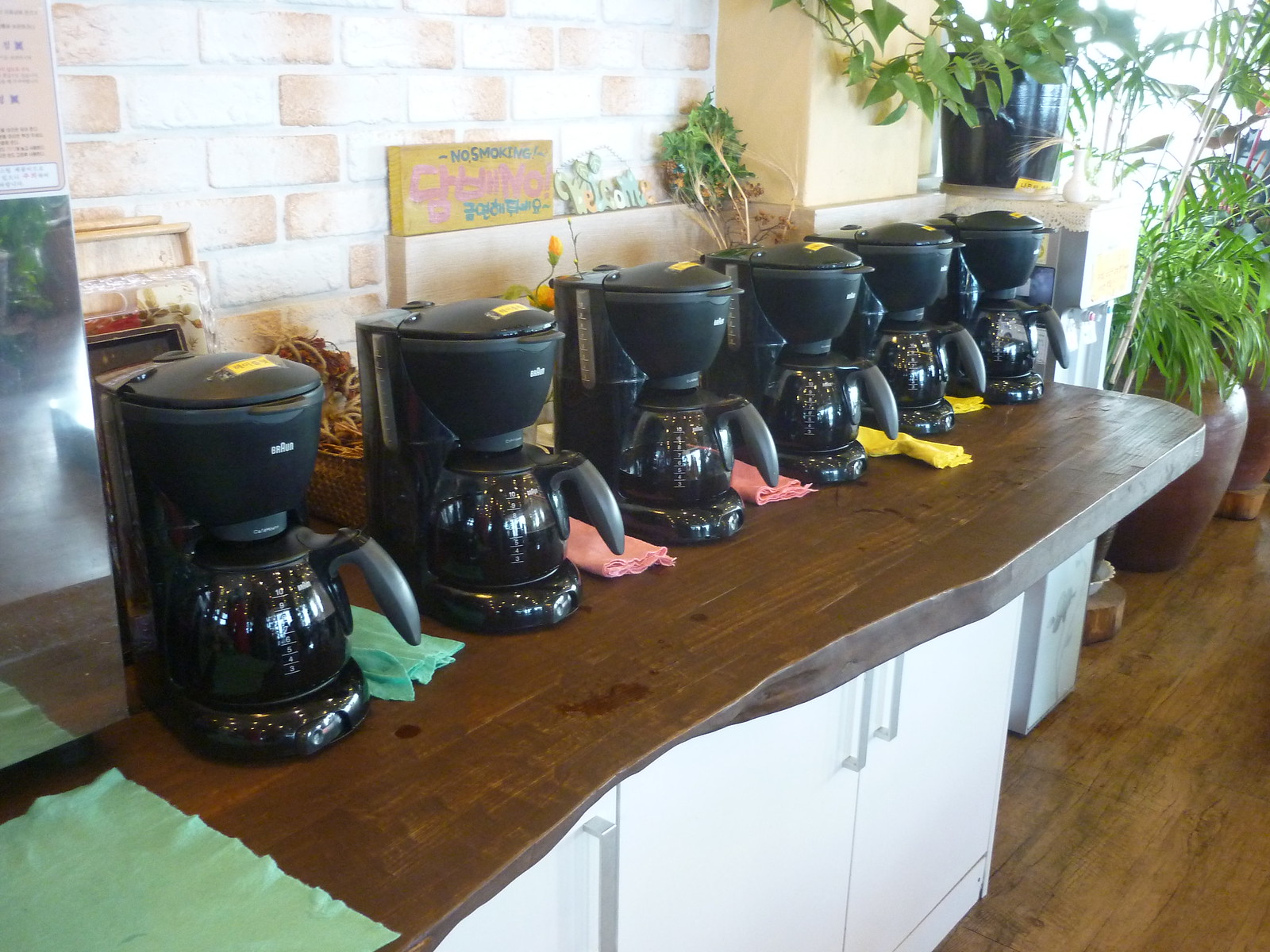In this detailed photograph taken inside a cozy café, a wooden counter hosts an array of six black 12-cup coffee makers, reminiscent of those often found at gas stations. Each coffee maker is labeled with yellow tags taped to the top, indicating the type of coffee within. The coffee makers are about three-fourths full and are accompanied by rags meant for cleaning spills; the towels come in various colors—green, pink, and yellow. Below the wooden counter, there are white cabinets adorned with silver handles, presumably for storage. The café's ambiance is enriched by lush, green climbing plants, both in black plastic planters on shelves and large terracotta pots on the hardwood floor. The backdrop features a charming brick-patterned wall, where a "No Smoking" sign is prominently displayed above the coffee setup.